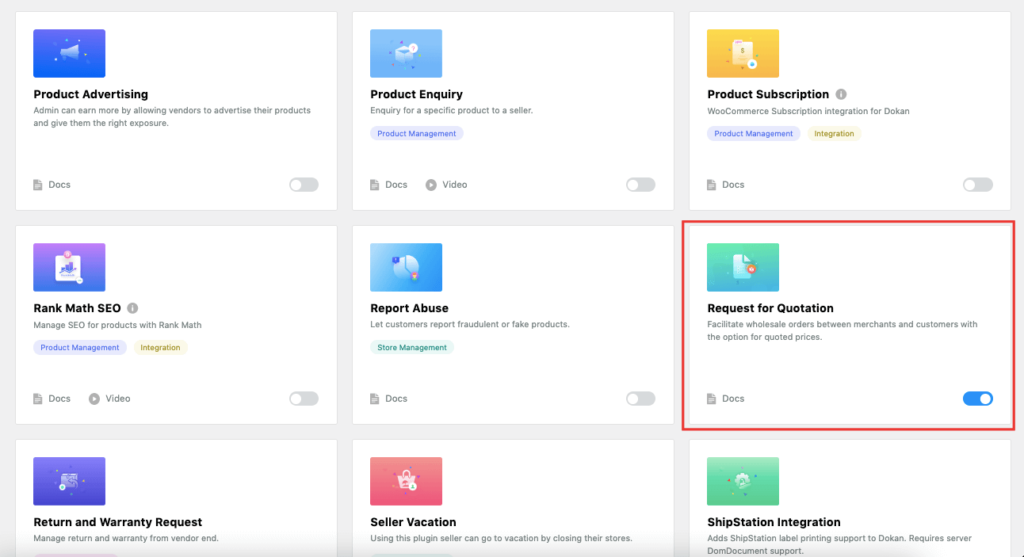The image features a gray background with a grid of nine white boxes arranged in three rows of three. Each box contains a link at the bottom labeled "DOCS." 

In the top left box, there is a blue square with text that reads "Product Advertising: Men can earn more by allowing vendors to advertise their product and give them the right exposure." 

The box in the top middle row is marked with the word "Video" in addition to the "DOCS" link at the bottom. 

The top right box is titled "Product Inquiry: Inquiry for a specific product to a seller."

Moving to the middle row, the left box also has "Video" above the "DOCS" link. 

The middle box in this row is labeled "Product Management."

The right box contains an orange square with the heading "Product Subscription: WooCommerce subscription integration for Dokan."

The third row has a blue box in the bottom left corner under which "RankMath SEO" is written. The remaining boxes adhere to the pattern of having the "DOCS" link at the bottom but lack additional labels or icons.

Overall, the image serves as a detailed directory or dashboard layout, with different sections highlighting various product-related functionalities and video resources.